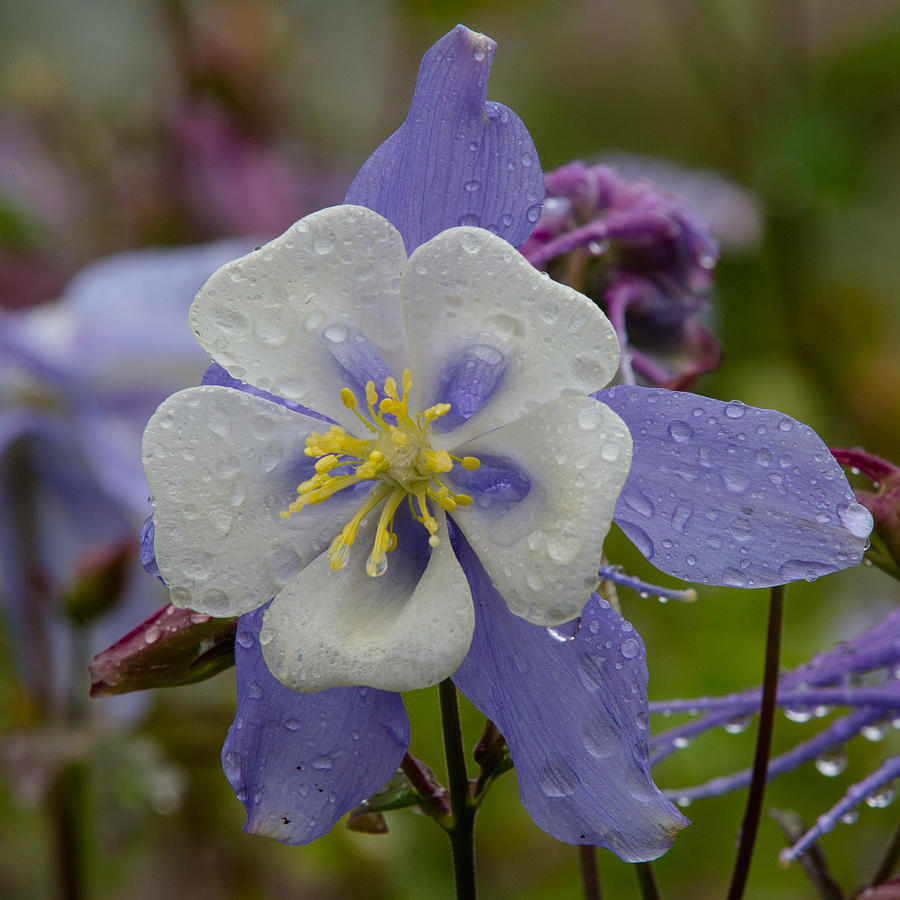This is a close-up photograph of a columbine flower, captured outdoors during the daytime. The flower, adorned with moisture from raindrops, showcases a striking combination of colors and textures. The outermost petals are a vibrant purple, arranged in a starfish pattern with five long and thin petals. In front of these, there are five large, floppy white petals with small purple ovals near their centers, which widen and round out towards the tips. From the heart of the flower, a dozen yellow stamens or pistils emerge, adding a splash of color and intricate detail. The dark reddish-brown stem beneath supports this vivid floral display. In the blurred background, other similar purple flowers are observable, alongside green foliage and even some dark maroon or reddish fuchsia blooms, creating a lush garden scene. The entire flower and its surroundings are lightly covered in glistening water droplets, emphasizing the freshness and natural beauty of this close-up shot.